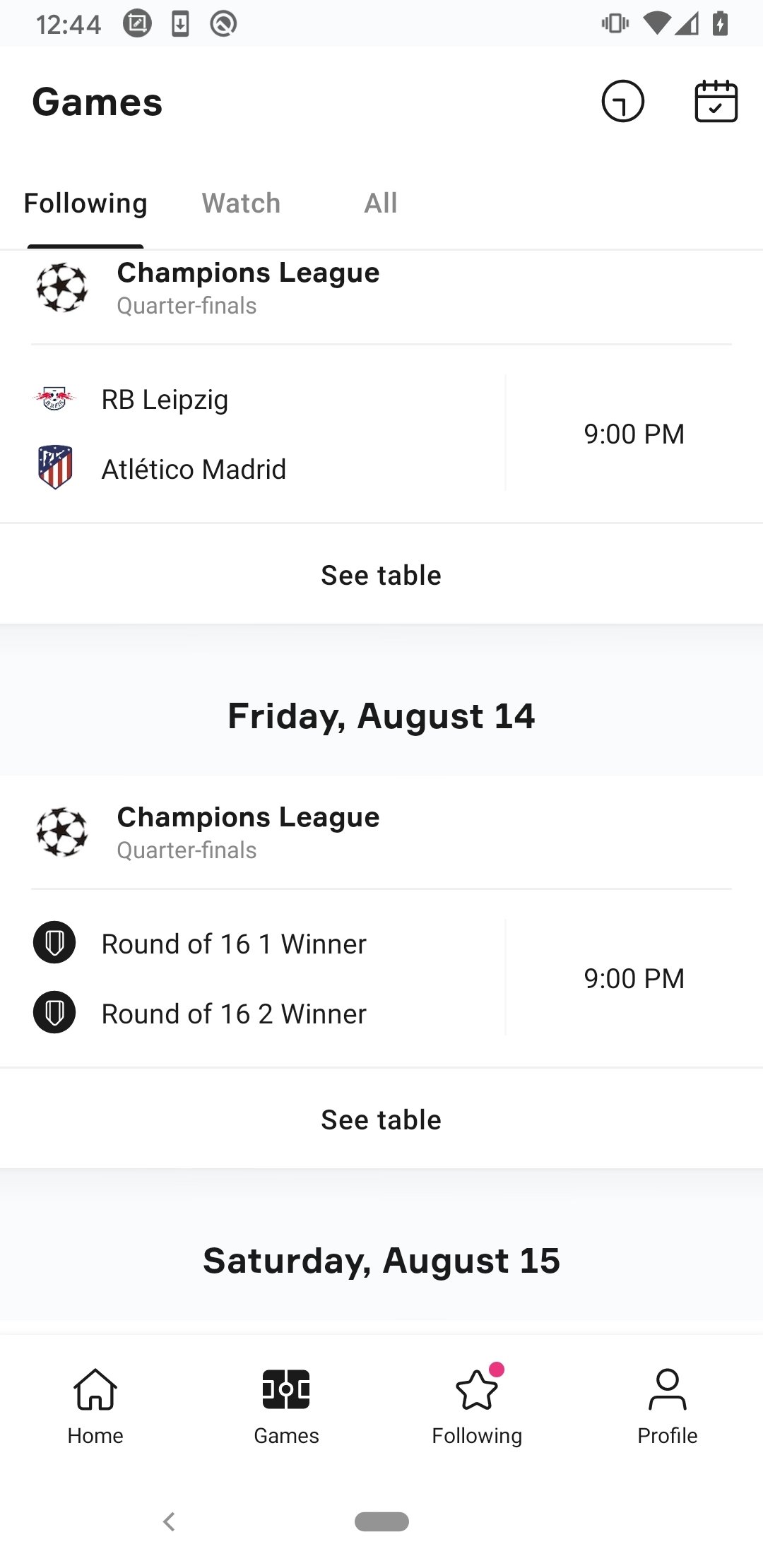This is a detailed screenshot from a smartphone, captured in a vertical orientation. At the top of the screen, the standard phone display information is visible, including the time, battery level, and signal strength. 

The primary focus of the screenshot is a "Games" page, indicated by the title at the top left. Adjacent to the title, on the right, are clock and calendar icons. Below this header, the screen is divided into three tabs labeled "Following," "Watch," and "All." The "Following" tab is currently selected, displaying events related to the user's followed teams.

The content under the "Following" tab shows a list of upcoming Champions League quarterfinal matches. Each entry provides specific details: the names of the competing teams, their respective logos, and the scheduled date and time of the matches. The text appears in a clear black font, ensuring readability.

At the bottom of the screen, a navigation bar offers quick access to various sections of the app, including "Home," "Games," "Following," and "Profile." Notably, the "Following" section has an active notification, indicating there are new updates or alerts for the user.

Overall, the screenshot effectively conveys a well-organized schedule of sports events, tailored to the user's interests.